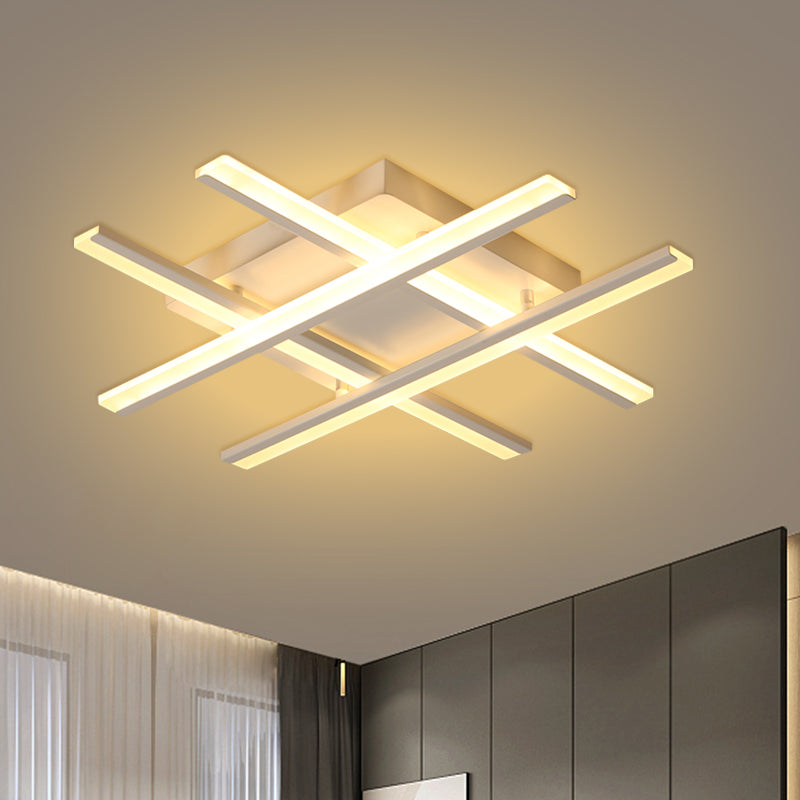The image captures a room, likely a bedroom or office space, with a strong focus on a unique ceiling light fixture. The fixture is a large, square design that resembles a hashtag or tic-tac-toe board, with four intersecting white wooden bars that each contain a light. The light fixture is directly attached to the ceiling, not hanging, and illuminates the room with a warm yellow glow. The background includes a wall, partially visible, colored dark green or black, and adorned with an art piece at the top. On the left side of the photo, there are windows covered with gauze curtains and darker, green curtains pulled to the side. The room appears dimly lit, further emphasizing the striking and creatively designed light fixture. The image does not include any text or writing.